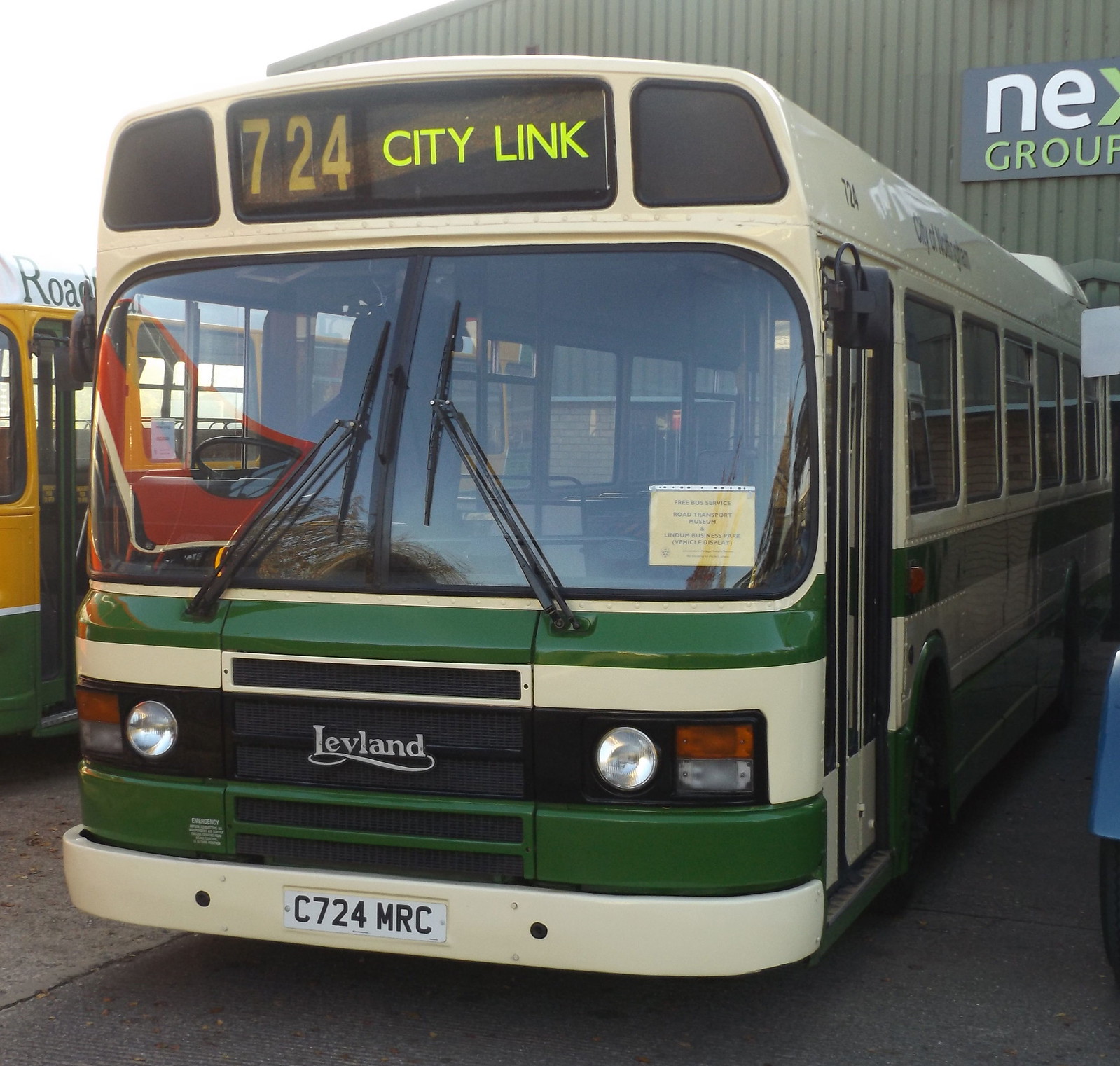This full-color daytime photograph, taken outdoors in Europe, features a parked city bus prominently in the foreground. The bus displays route number 724 and the destination "CityLink" on a digital display at the top. It is adorned in green and cream/white colors, with a green and white alternating stripe design and a European-style license plate reading C724MRC. The make of the bus is Leyland, marked in silver on the grill. A large windshield occupies the front, with wipers positioned upright, and the bumper is cream-colored. The bus is parked on a concrete surface with a noticeable crack, and there is no one inside.

In the background, a gray corrugated metal building with a partial sign reading "NEX Group" is visible. Another bus, with a white top, yellow middle, and green bottom, is partially seen to the left of the main bus. The scene's composition suggests an urban or industrial setting, with the bright sunlight shining from the upper left corner, highlighting the daytime context.